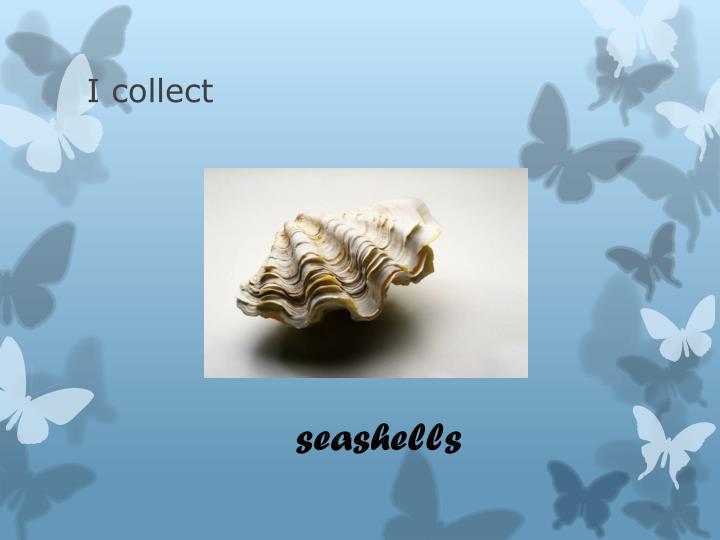This image features a card with a serene, light blue background adorned with delicate butterfly silhouettes in shades of blue, light gray, and white, arranged along the left edge, the right edge, and the bottom right corner, gradually extending towards the center. In the top left corner, the phrase "I collect" is printed in thin black letters. Dominating the card's center is a photo of a seashell set against a light gray backdrop. The seashell showcases a textured surface with distinctive undulating patterns and striations in shades of white, brown, and dark yellow, casting a prominent dark shadow beneath it. Positioned below the seashell photo, the word "seashells" is boldly written in thicker, larger black letters.